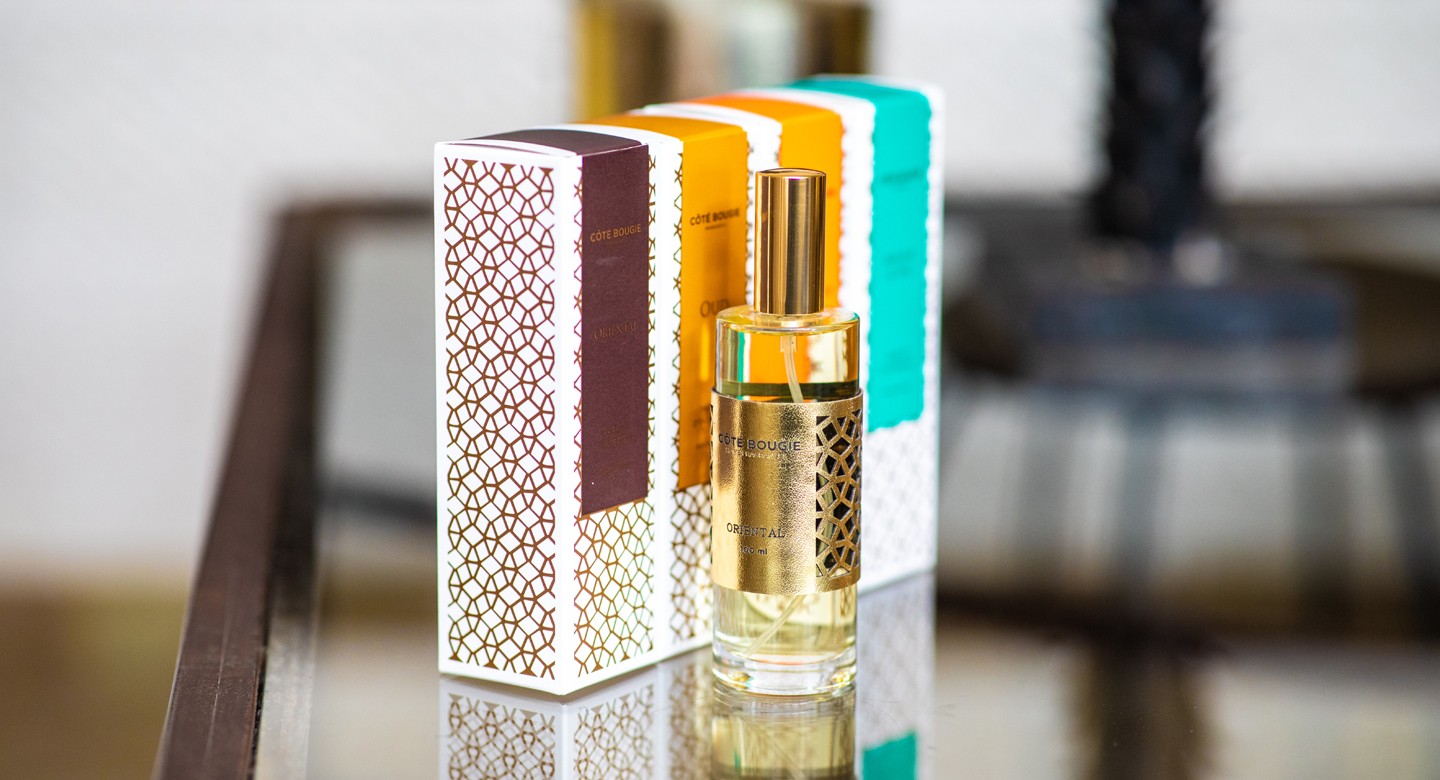This indoor, staged photograph features a perfume bottle and its packaging. The central focus is a clear glass bottle containing a transparent liquid, equipped with a spray top and adorned with an indistinguishable gold label. Surrounding the bottle are four vertically rectangular boxes, resting on a glass-top table with a brown wooden frame. The boxes, presumably of the same brand, feature distinctive stripes: one with a burgundy stripe, two with gold stripes, and one with a turquoise stripe. The background includes a white wall, and the slightly blurry image hints at a possible lamp base on the table and wooden flooring.